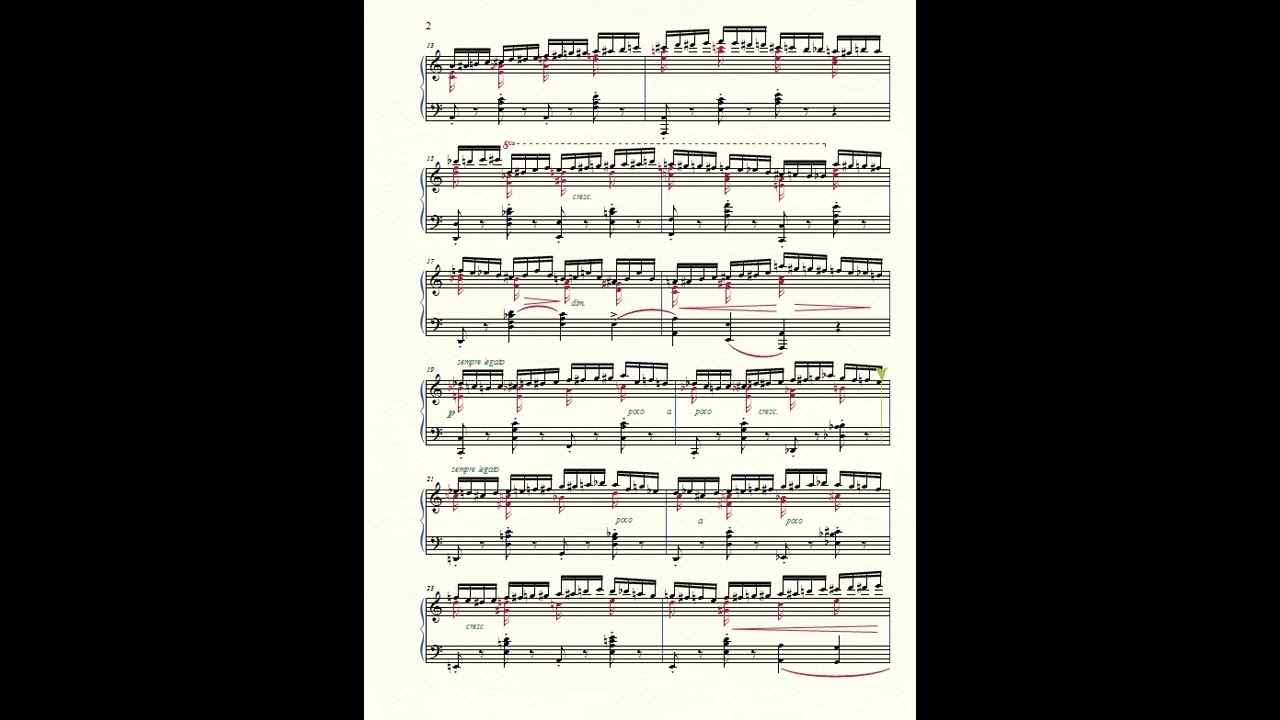This image captures a scanned, black-and-white sheet of music framed by black borders on the left and right sides. The music sheet, marked as page two, is adorned with a mix of treble and bass clefs, suggesting it may be arranged for piano or a similar instrument. High notes dominate the top of the staves on the treble clef, while sparse lower notes appear on the bass clef. The upper part of the sheet features numbers in sequence — 15, 13, 15, 17, 19, 21, 21 again — accompanied by the phrase "Semper Legato." Red markings and notes are scattered throughout the sheet, adding a distinctive visual contrast to the monochrome background. No title or additional text is visible, and there are no people in the image.